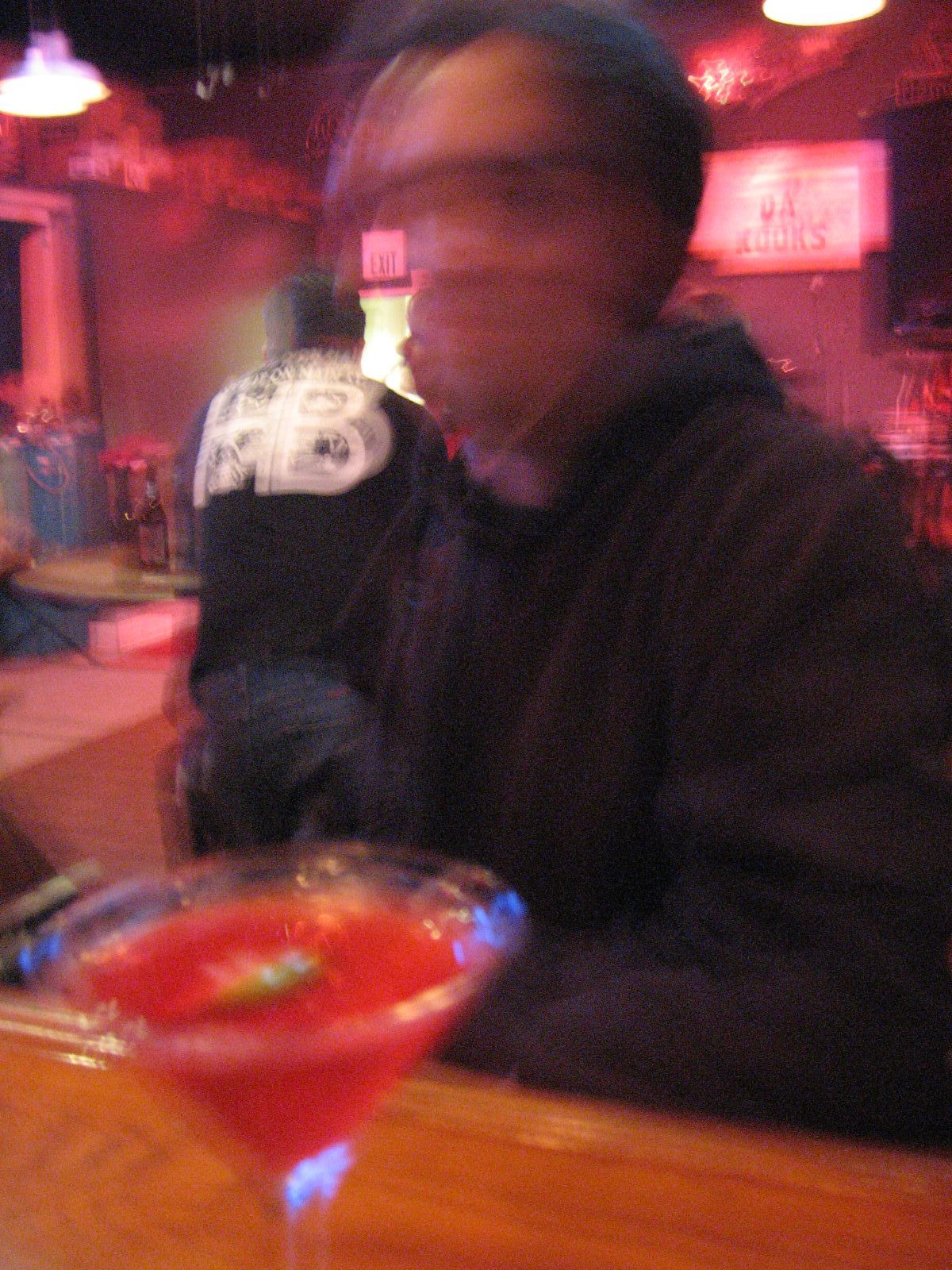In this extremely blurry photograph of a bar interior, a man in the foreground is seated at a wooden counter, wearing a black hoodie or sweatshirt. His face is highly blurred, with only his left eye somewhat discernible, giving an impression of anonymity. In front of him rests a dark pink drink, possibly in a daiquiri or martini glass, garnished with what appears to be something green or yellow.

Just behind him stands another man in a black shirt featuring the letters "HB" in white text on the back, paired with blue jeans. The bar area around them is illuminated by a red light that highlights a pink wall in the background. Various beer bottles and a white exit sign are visible near the second figure. Adding to the scene's ambient details, a "Da Cooks" sign on a white background is situated to the right of the seated man's head. From the ceiling, a few lights hang, casting a warm glow on the overall setting. Despite the photograph's lack of focus, these elements collectively paint a vivid picture of a lively bar scene.